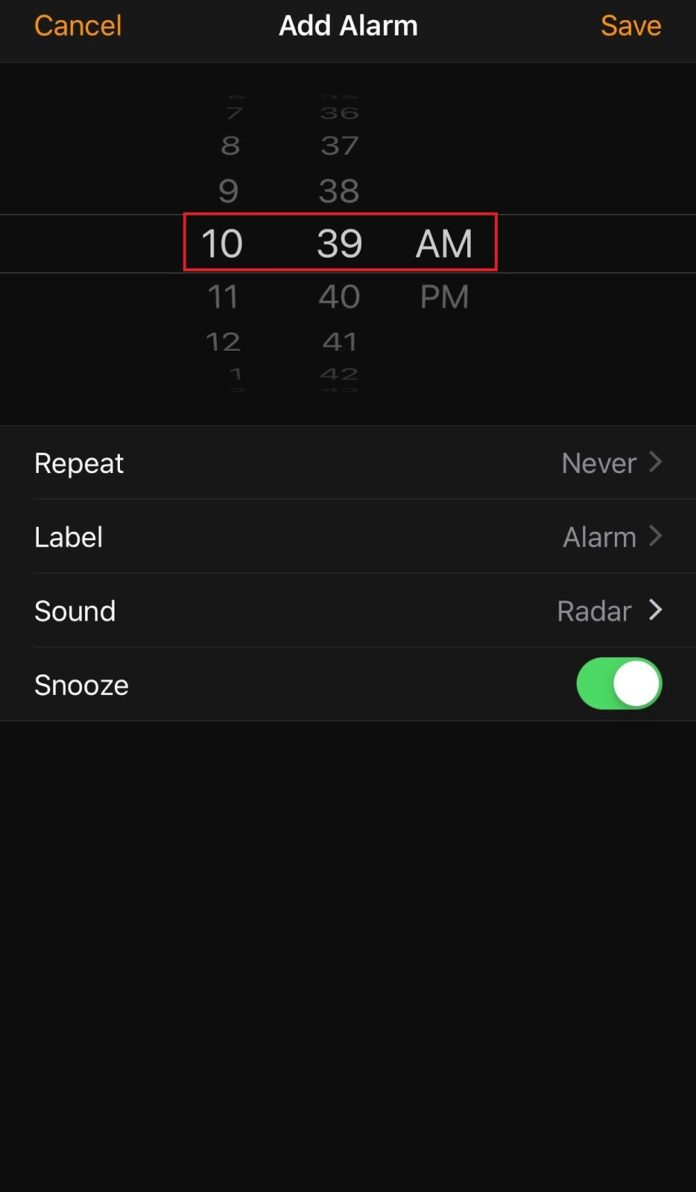A digital clock displays the time as 10:39 a.m. The interface showcases several buttons labeled "Repeat," "Never," "Label," and "Sound Radar," alongside options to "Snooze," "Toggle," "Cancel," "Add Alarm," and "Save." A series of times is listed below: 9:38, 8:37, 7:36, 11:40, 12:41, and 1:42 p.m. The background is dotted with thematic icons related to household, children, deliveries, school research, training programs, and various school policies, including continuity, prevention, generation, tradition, community learning, and data management. The intricate design reflects a meticulous organization of daily routines and academic regimes.